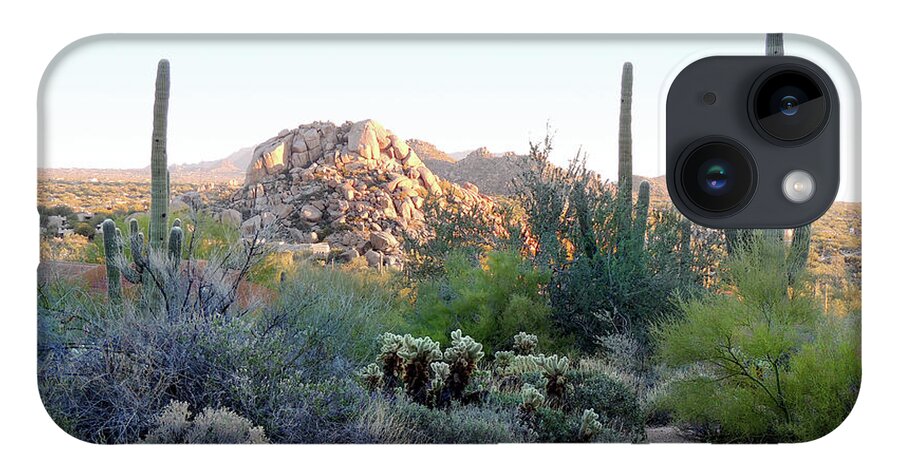This image showcases an iPhone laying horizontally, displaying its distinctive dual-lens camera setup on the top right within a square module, accompanied by a microphone and a flash. The phone case features a panoramic desert landscape with a prominent rocky hill in the background under a clear, sunny sky. The foreground is adorned with various succulent plants, including three tall cacti—one on the left and two on the right—alongside smaller bushes and green foliage. The scene is devoid of animals, emphasizing the stark, arid beauty of the desert terrain.